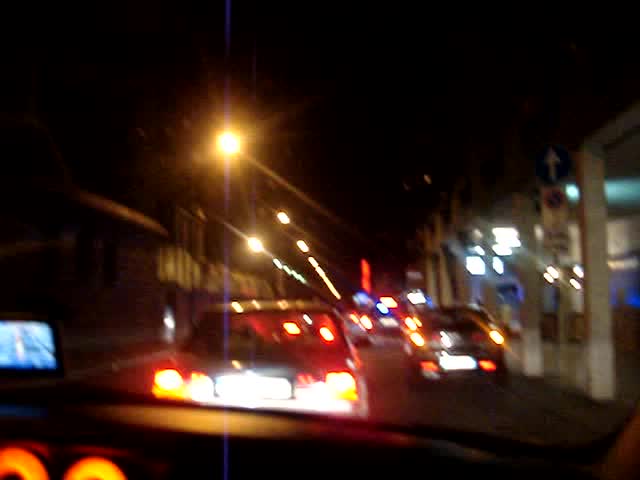The photo captures a view from the passenger seat of a car, looking out through the windshield onto a moderately trafficked road at night. On the left side of the road, there are rows of houses, while the right side features a parking deck. The scene is dimly lit by street lights, which create a glare in the upper part of the image. Inside the car, a GPS device with an illuminated LED screen is visible on the left side of the dashboard. Additionally, the dashboard indicators cast a faint glow, adding depth to the interior perspective.